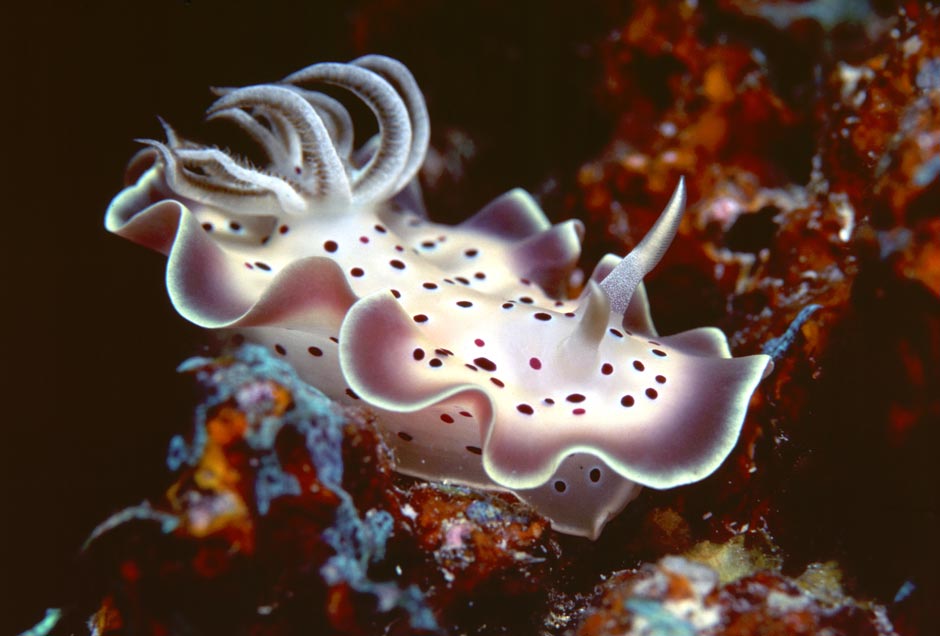This underwater photograph captures the fascinating sight of a nudibranch, a type of sea slug that inhabits the deep ocean. Positioned diagonally in the center of the image, the nudibranch is predominantly white with light pink scalloped edges, accentuated by dark red and magenta polka dots across its body. The creature features tentacle-like appendages protruding from its top and back, giving it an otherworldly appearance. It rests upon or swims near brightly colored orange or dark red plankton or sea coral, set against the background of the deep, dark ocean depths. The surrounding environment also includes red barnacles, adding to the vibrant yet eerie underwater scene typically encountered by scuba divers. The overall mood of the photograph is mysterious, highlighting the bizarre and intricate beauty of deep-sea life.